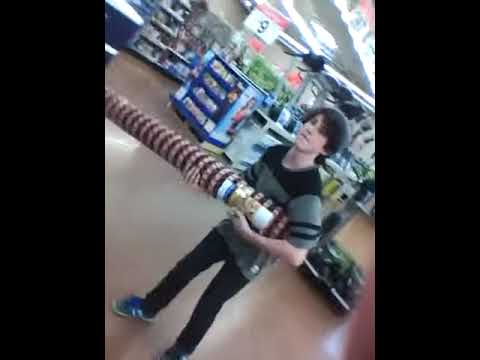Inside a Walmart department store, two young men, possibly teenagers or in their early 20s, are captured engaging in what looks like an impromptu sword fight using rolled-up rugs. The photo, originally taken in portrait mode but displayed in landscape, reveals these individuals playfully positioned in an aisle with numerous items and price signs in the background. 

The shelving units in the background display various items, including a stack of blue coolers with white lids. One young man, with black hair and wearing a gray beanie, has on a black and gray shirt paired with black pants. He is holding a reddish-tan checked rug that stands on the floor. The other young man, who has blonde hair, is dressed in a blue shirt, black pants, and gray shoes; he is mid-action, pointing a gray rug toward his friend. Both rugs still have their labels attached. Displays behind them include price signs with numbers like $52, 97, and 2, hinting at their location amidst the store's low price promise, possibly near the electronics or camping section. The floor beneath them appears to be brown linoleum or tile, adding to the classic department store ambiance.